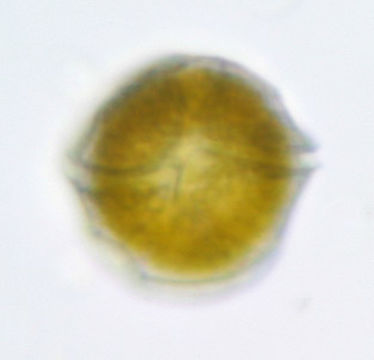This image displays a highly blurry and pixelated hand drawing against a light steely gray background. The central subject resembles a walnut or round-shaped object with poorly defined edges, drawn in black. The object itself appears brown to gold with the inner areas becoming lighter toward the center, transitioning from gold to light yellow to white. Ridges or creases run along the center and top, giving it a somewhat tubular, bagel-like appearance. Despite the blurriness obscuring many details, the image also hints at a resemblance to algae or possibly a microscopic organism, suggesting it might have been taken in a lab setting. The overall quality loss and foggy edges contribute to the difficulty in identifying the object definitively.